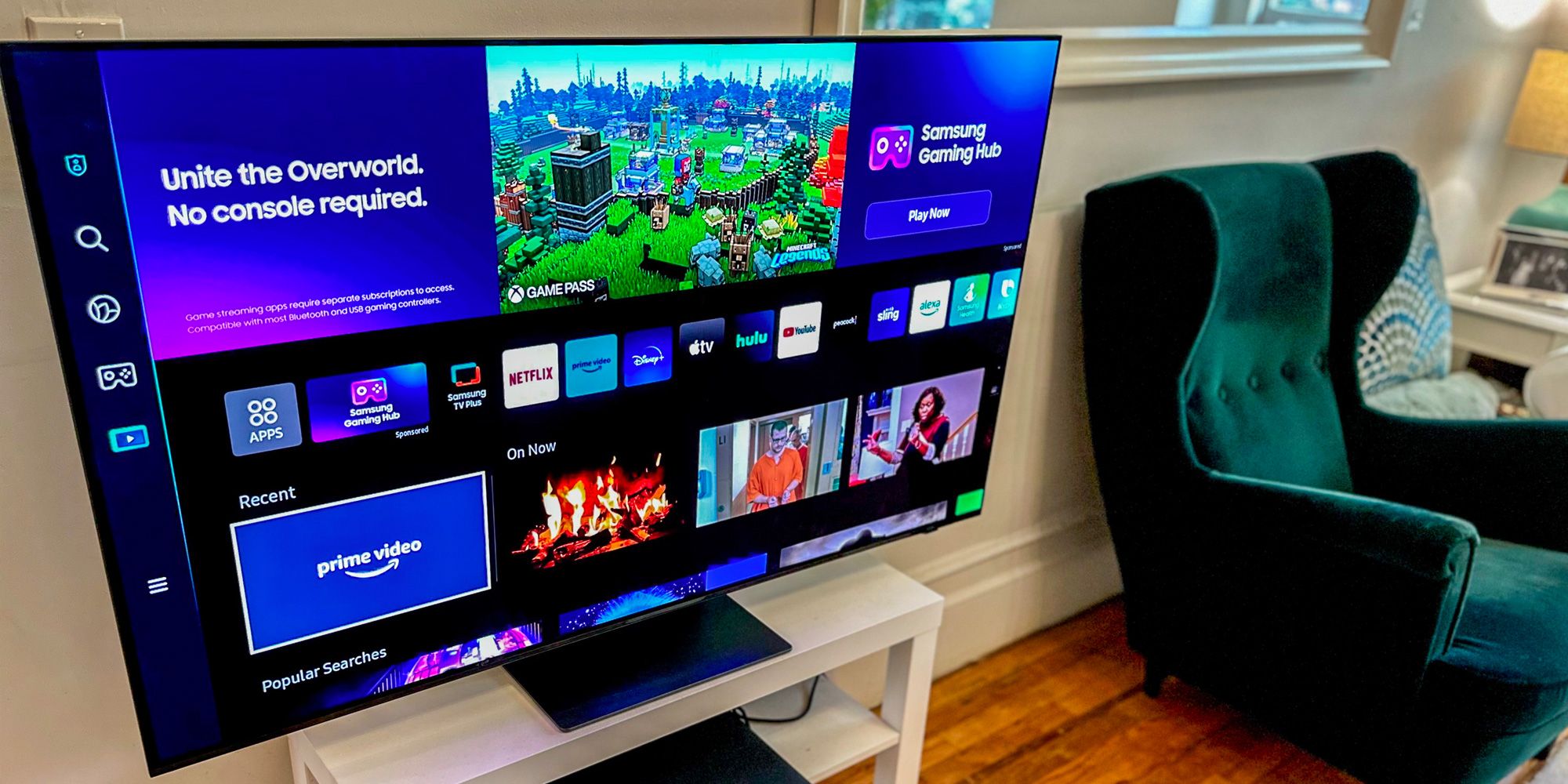The image depicts a cozy living room or den with a central focus on a Samsung smart television, dominating the left three-fourths of the picture. The TV is mounted on a small white stand and displays its home screen, featuring various apps like Netflix, Prime Video, Disney+, and Apple TV, with recognizable Samsung branding and interface elements. The hardwood floor, neither too dark nor light, complements the white walls and lends a warm atmosphere to the room. To the right of the TV is a comfy dark green, velvet single-person lounge chair. Beside the chair, partially cut off at the corner, is a small white table with a lamp and a photograph. Above the chair, there is a mirror that enhances the room's decor. The setup suggests a welcoming and functional living space, perfect for relaxation and entertainment.